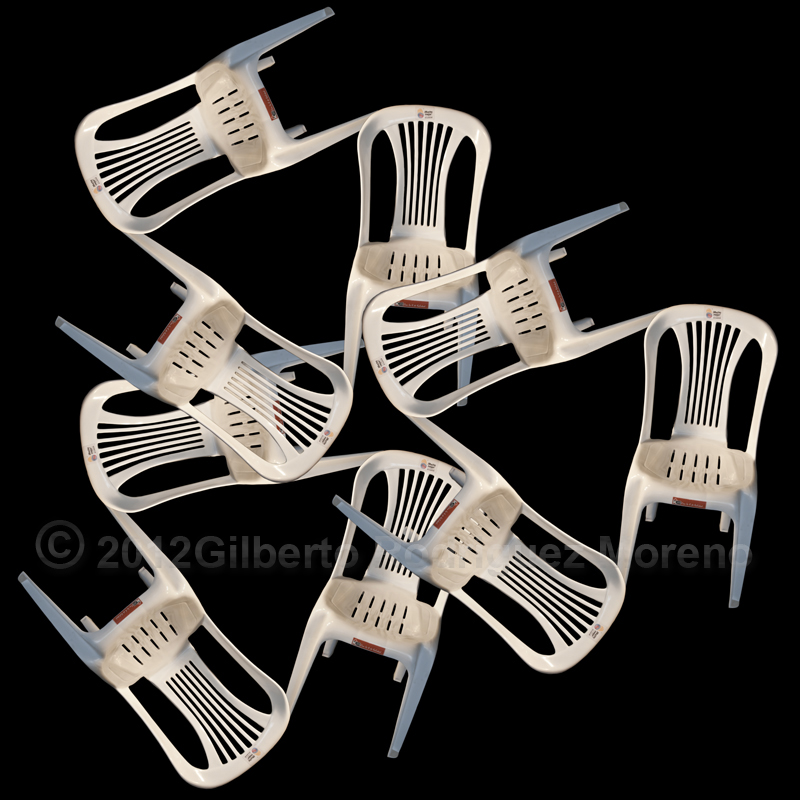The image showcases nine white, molded plastic lawn chairs without armrests, each with the right front leg in a gray hue. The chairs have a fan-like back configuration featuring five interior stripes and solid areas on the sides. The seats are solid, punctuated by two rows of five slits. The arrangement appears chaotic, with chairs positioned at various angles on a black background, giving an impression of them flying or floating. A watermark reading "Copyright 2012 Gilberto" is partially visible across the front, suggesting the image could be a computer-generated digital artwork or a stock photo.